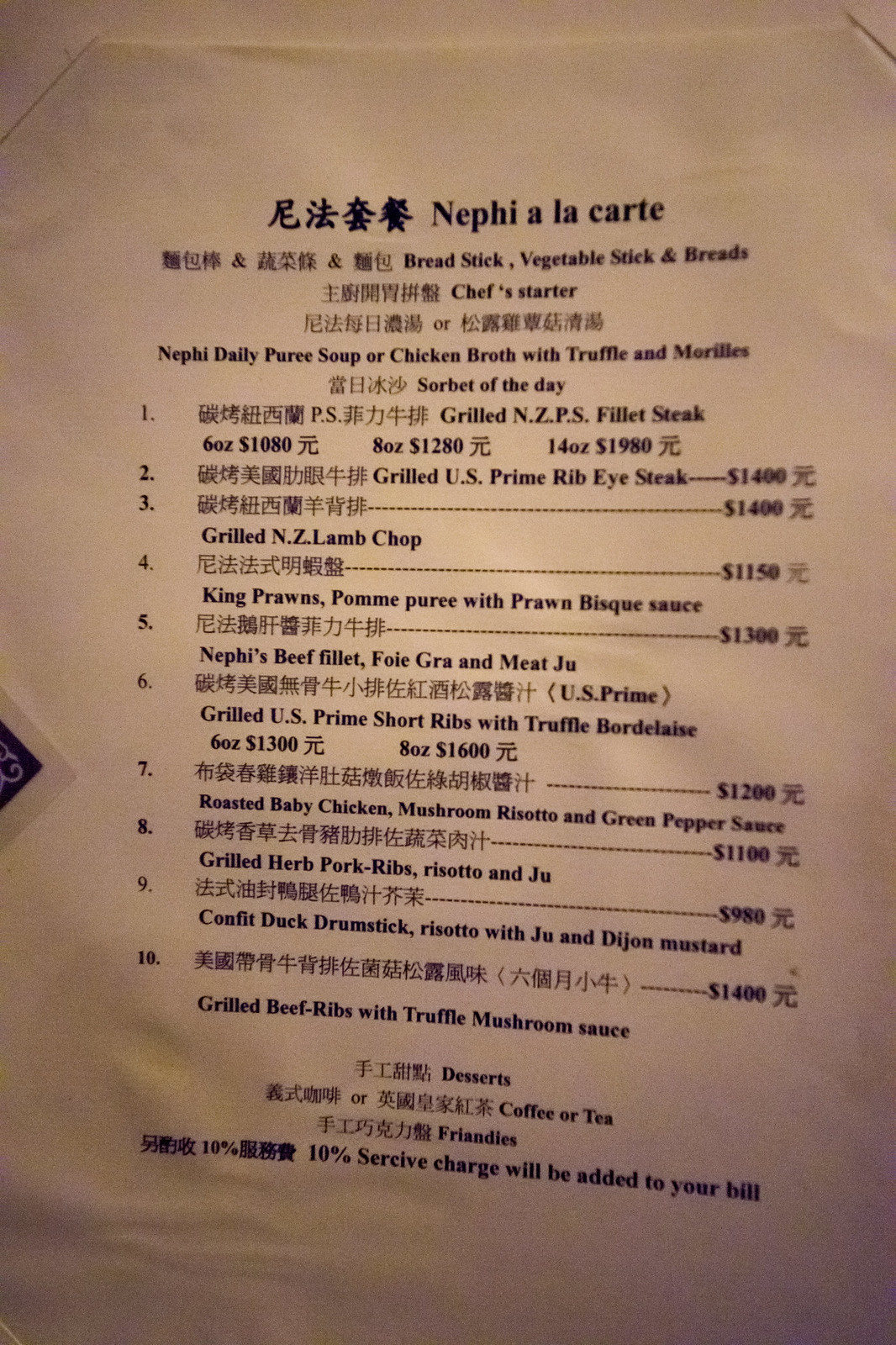This photograph features a menu presented on a small piece of white paper, printed entirely in black ink, giving it a clean, monochromatic aesthetic. At the top of the menu, there are Asian characters, followed by the title "Nepi a la carte." Beneath the title, more Asian characters appear in a smaller font size. 

Directly next to these characters, in English, the menu lists "Breadstick, Vegetable Stock, and Breads." Below this section, the image becomes slightly blurred, compromising the picture quality, yet the text "Chef Starter" is still discernible in English, accompanied by more Asian characters. Further down, the menu states "Nepi Daily Puree Soup or Chicken Broth with Truffle," although the words next to it are too blurry to read clearly.

Following these descriptions, the menu transitions into a numbered list of main courses, labeled from 1 to 10, each accompanied by a price. Despite the use of the dollar sign, the high prices suggest the currency is not U.S. dollars. For instance, the first entrée, a "Grilled U.S. Prime Ribeye," is priced at $1,400. At the very bottom, the menu highlights the availability of desserts, coffee, or tea, and notes a 10% service charge.